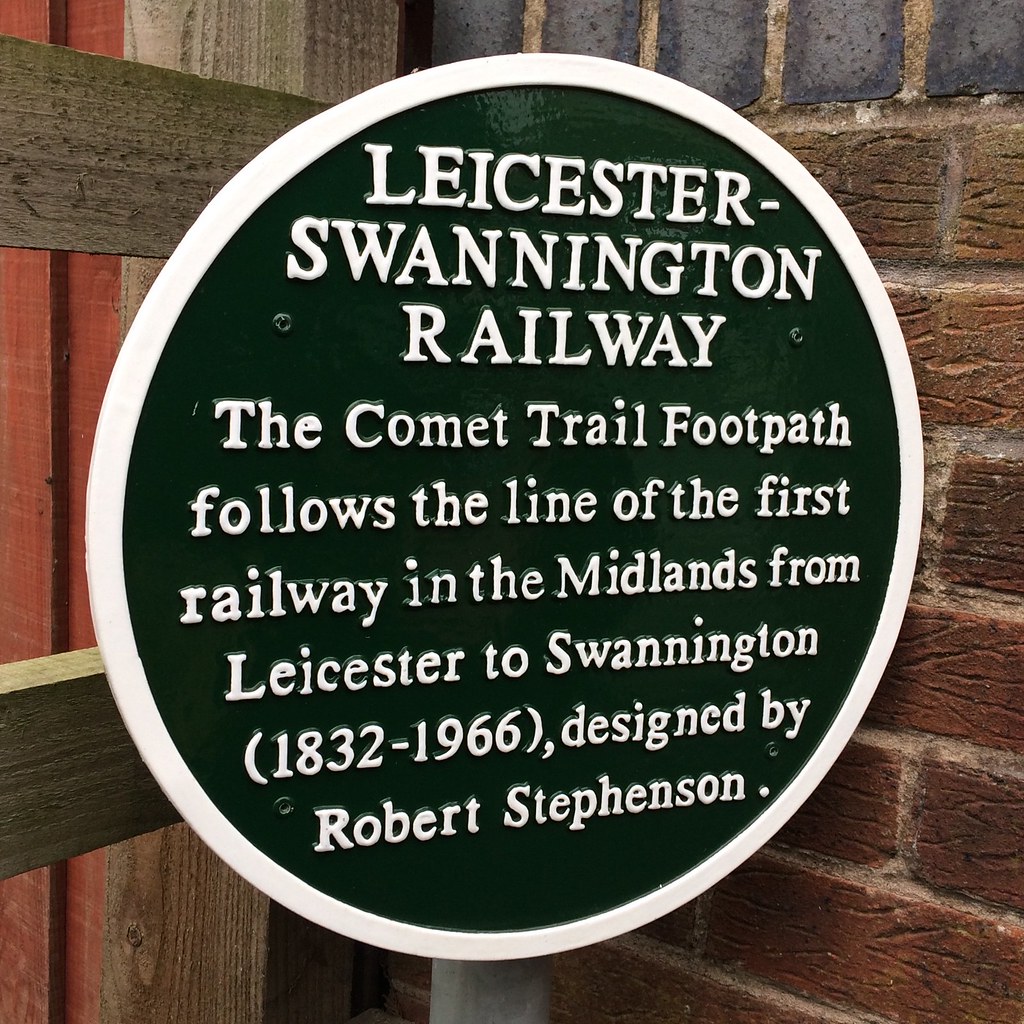The image depicts an outdoor scene centered around a round sign with a white edge and black center, featuring white lettering. The top of the sign prominently displays "Leicester-Swannington Railroad" in large, all-caps font. Beneath it, in smaller print, the sign reads: "The Comet Trail footpath follows the line of the first railway in the Midlands from Leicester to Swannington, 1832 to 1966, designed by Robert Stevenson." The sign is set at the intersection of a wooden fence and a brick wall. The fence to the left features horizontal and vertical wooden slats, with some natural wood-colored and others painted red. The brick wall behind the sign is composed of red bricks, transitioning to dark black bricks at the top. The photograph likely captures an overcast day, as there are no visible shadows or distinct lighting effects.